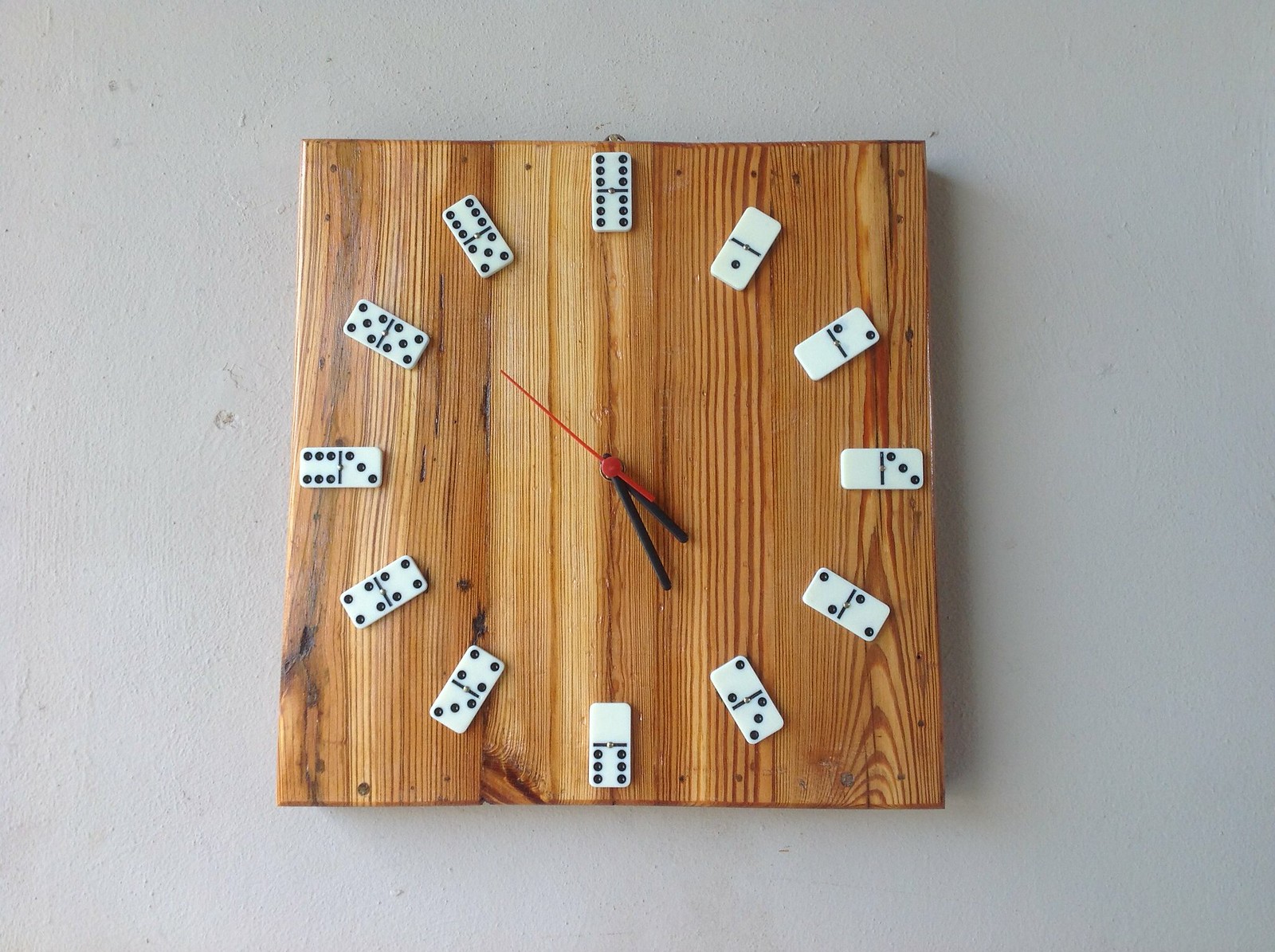This image portrays a uniquely handmade clock crafted from a piece of wood, either rectangular or square, showcasing its natural grain and various shades of light brown. Prominently featured are the visible wood grain and knots, adding to its rustic charm. The clock's hands are a stark black, contrasting with the singular red second hand. What sets this clock apart is its creative use of dominoes for the numerals; each number from one to twelve is represented by white dominoes adorned with the corresponding number of black dots. These dominoes are securely affixed to the wooden background. The clock is mounted on a plain white wall with a visible screw at the top, giving it a simple yet intriguing aesthetic.